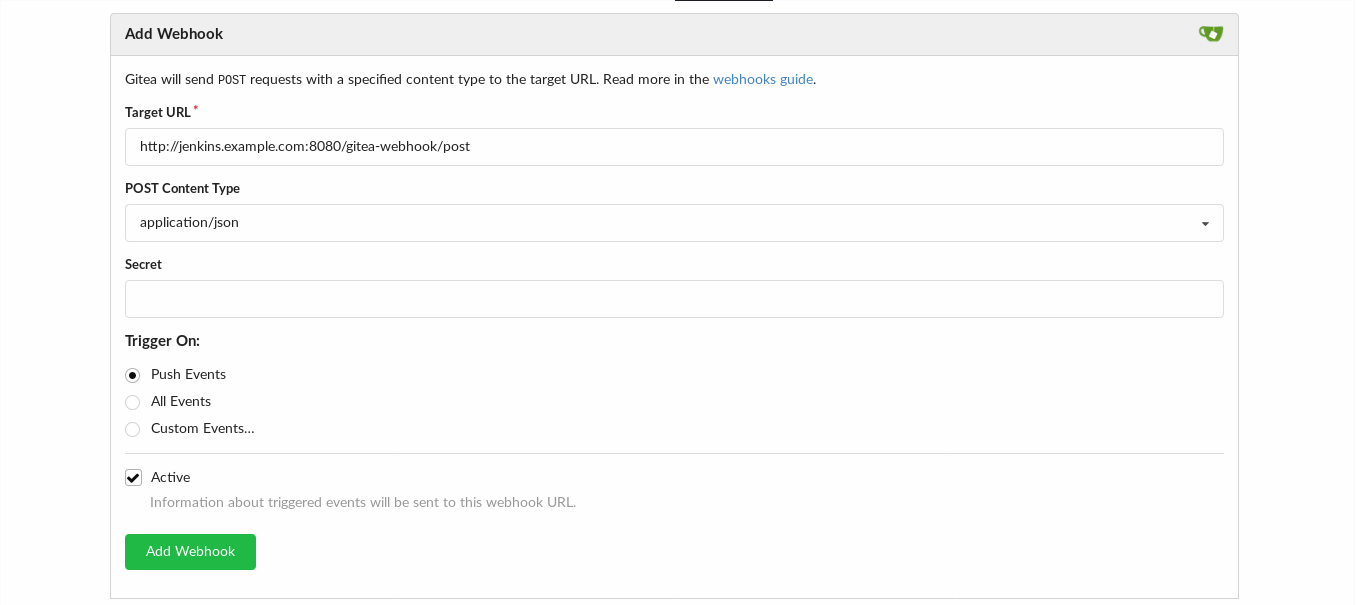**Detailed Caption:**

The screenshot captures the interface for adding a webhook in Gitea. At the top, the title bar reads "Add Webhook" in bold black font against a light blue background. Below the title, a description explains that Gitea will send POST requests with a specified content type to the target URL, followed by a clickable blue link labeled "Webhooks Guide."

The main content showcases several configuration options. The target URL field contains a partially obscured URL: "http://jenkins.example.com:8080/Gitea-webhook/post." Following this, the "Post Content Type" field specifies "application/json." An empty text box is provided for a secret.

The "Trigger On" section offers three radio button choices: "Push Events" (selected by default), "All Events," and "Custom Events." Below this, there is a checkbox labeled "Active" which is checked, indicating that information about triggered events will be sent to the specified webhook URL.

At the bottom of the form, a prominent green button labeled "Add Webhook" is positioned, ready to execute the webhook addition.